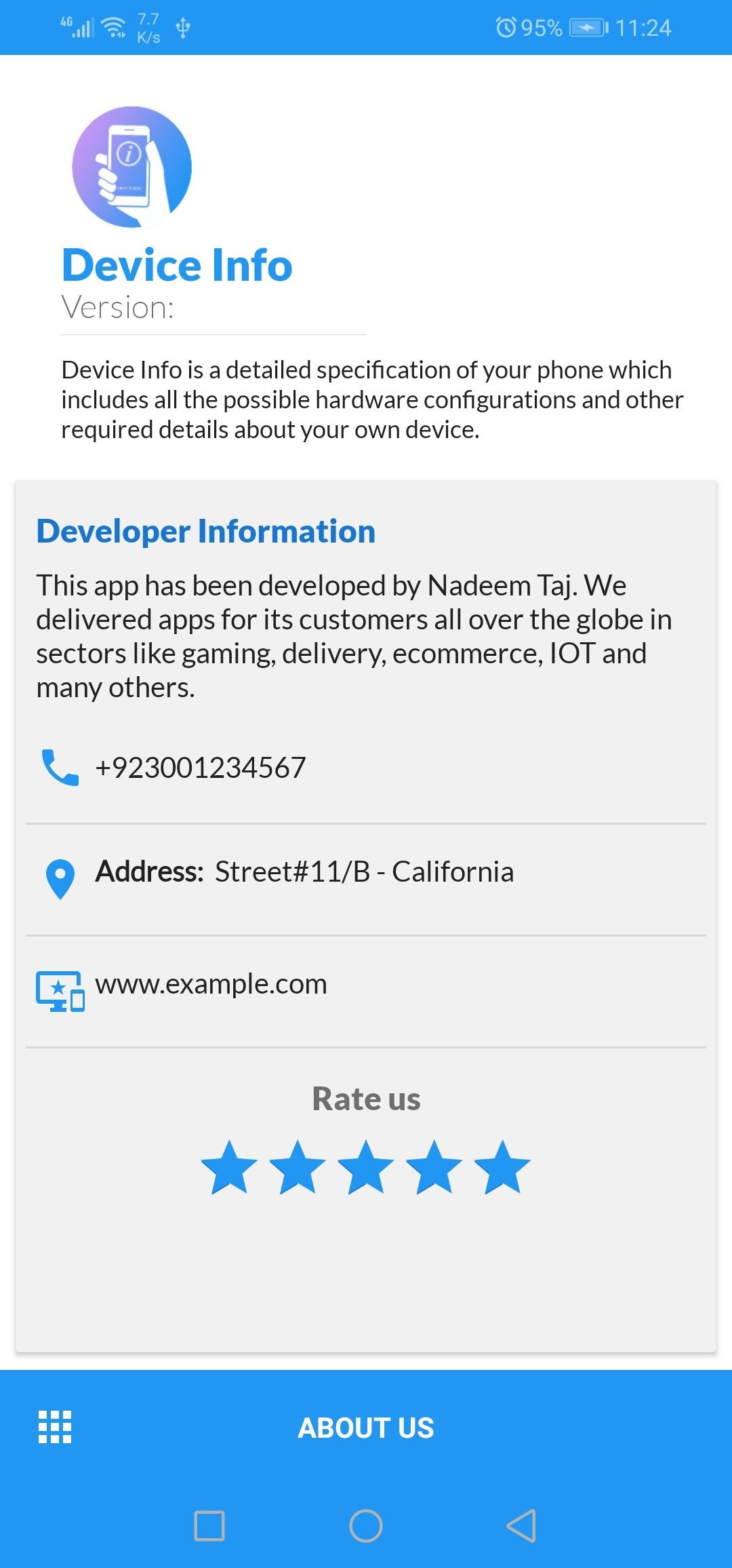**Detailed Screenshot Caption:**

This screenshot is taken from a smartphone, displaying detailed device information. The top and bottom borders of the screen are highlighted in blue. At the upper left corner, there is a round icon depicting a hand holding a cell phone, enclosed within a circle that blends blue and purple hues. Beneath this icon, the text "Device Info" is presented in blue. The subsequent line, in gray text, shows "Version:" followed by a thin gray horizontal line stretching halfway across the screen. Below this line, in black text, it reads: "Device info is a detailed specification of your phone which includes all the possible hardware configurations and other required details about your own device."

The background below this section transitions to gray. In blue text, "Developer Information" is shown. The following line in black text states: "This app has been developed by Nadim Taj. We deliver apps for customers all over the globe in sectors like gaming, delivery, e-commerce, IoT, and many others." Adjacent to a blue telephone icon, the contact number is displayed in black as "+92 300-1234567."

A further thin gray horizontal line crosses the screen. Next, a blue location icon is shown, with the address "Street number 11/B, California" written in black text to its right. Another thin gray horizontal line follows. Subsequently, a blue computer icon, overlaid with a blue smartphone, appears to the left, and the website "www.example.com" is listed in black text to its right. A final thin gray horizontal line is drawn across the screen. At the bottom center of the screenshot, the text "Rate Us" is displayed in black, and directly below it, there are five blue stars aligned in the center of the page.